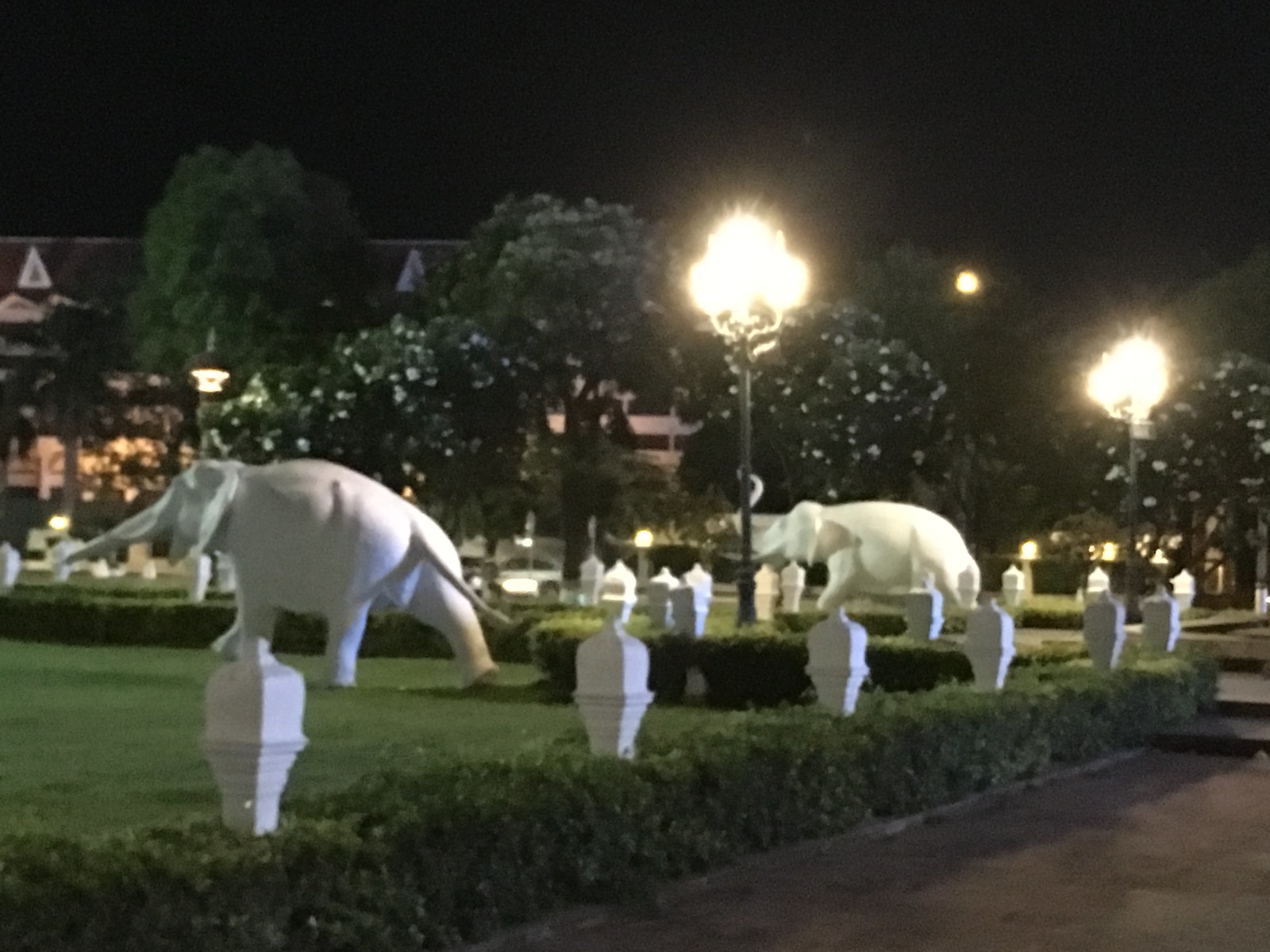The photograph captures a serene nighttime scene in a well-maintained park. Dominating the foreground are two life-sized white elephant statues with artistic, glossy surfaces, perhaps made of marble or alabaster. One elephant has its trunk raised high, while the other extends its trunk forward. They stand on a meticulously manicured grassy area, enclosed by well-trimmed shrubs that are bordered by illuminated white posts. The surrounding park features a gray walkway, flanked by lush green bushes. Bright street lamps with black posts vividly light up the area, adding to the inviting ambiance. In the background, a large estate or building is partially visible, shrouded by tall trees, hinting at an affluent and secure environment. The overall atmosphere suggests a warm, welcoming place perfect for an evening stroll.